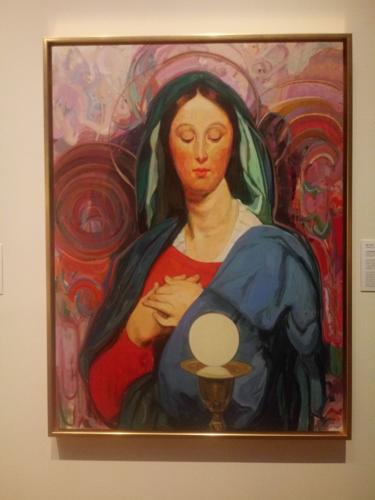This detailed painting, framed in a reflective brownish-golden frame, captures the serene image of a woman from head to waist, hanging prominently on a white-walled space, likely in a home, art gallery, or museum. The woman, with her pale complexion and reddish-brown, middle-parted hair, wears a blue robe over a red dress. Her head is adorned with a teal hood with a light-green lining. Her hands are clasped over her chest, albeit with the left thumb incorrectly placed underneath the right hand. She gazes down at a golden chalice that holds a glowing, orb-like object, reminiscent of a crystal ball. The background of the painting is an abstract swirl of pink, red, violet, purple, orange, and gold tones, which form a halo-like effect around her head and add to the overall mystical and artistic impression.